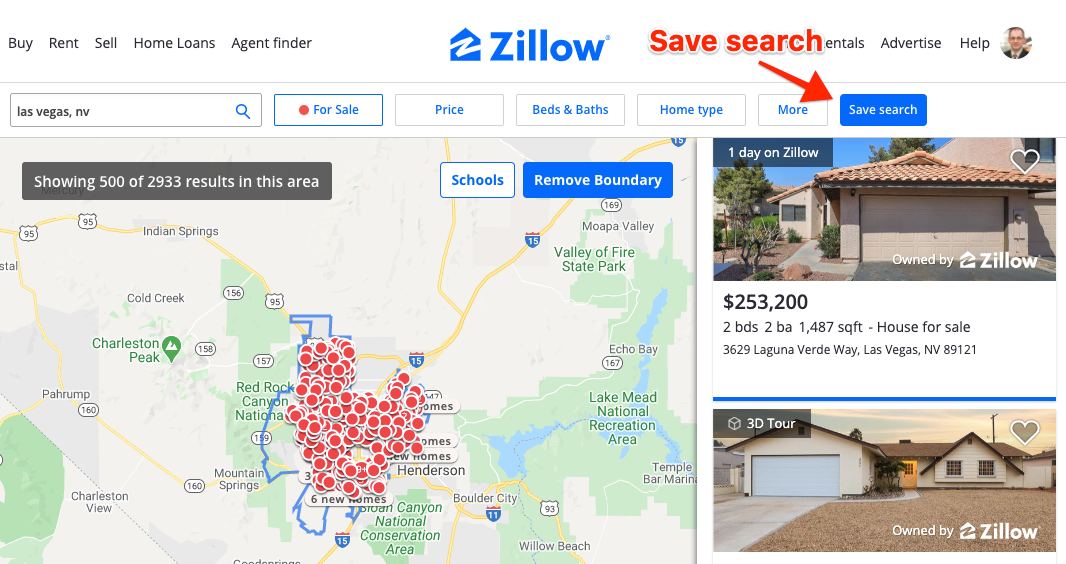This image is a screenshot of a Zillow webpage, prominently displayed in the center of a white background. The Zillow logo, featuring blue text and a house graphic with a white 'Z' through it, stands out. At the top of the page, several tabs are visible: "Buy," "Rent," "Sell," "Home Loans," and "Agent Finder." 

An overlay graphic with a large red arrow and the text "Save Search" directs attention to the blue "Save Search" button on the page. In the upper right corner, a profile icon of a man wearing glasses, a white button-down shirt, a black coat, and a tie can be seen. 

The search parameters are set for properties in Las Vegas, Nevada, as indicated in the search bar next to a blue magnifying glass icon. The top section of the search results displays various filters: "For Sale" marked with a red dot, "Price," "Bed & Bath," "Home Type," "More," and the crucial "Save Search" button. Below these filters, two property listings are partially visible. One of the homes is listed at a price of $253,200 and spans 1,487 square feet.